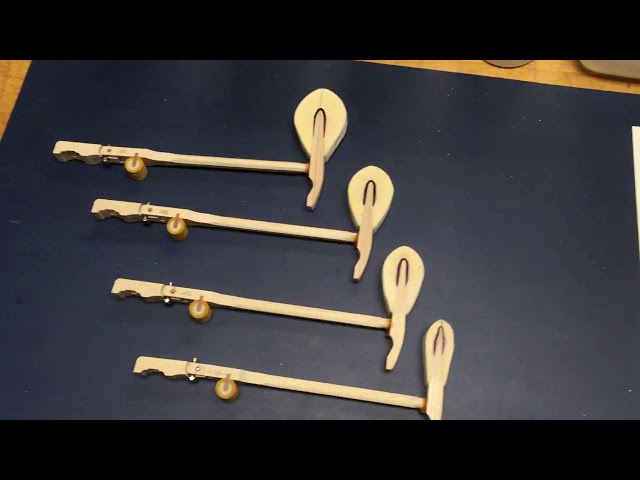The image showcases a series of four hammers, which have been removed from the inside of a piano. These hammers are arranged vertically, from top to bottom, in decreasing order of size, while maintaining the same length. They are meticulously constructed from light-colored wood and feature a small divot on the left side near the bottom. Approximately a couple of inches above the divot, a cylindrical roller or pivot point is attached. Each hammer is oriented at a 90-degree angle to the lever part, which is a straight section of wood. The tips of the hammers are wrapped in a small piece of dark fabric, followed by a larger piece of white padding, which is the striking surface used to hit the strings. The hammers are laid out on a black background, emphasizing their detailed construction and the subtle gradients in their wood tones. Their carefully arranged positioning and descending size create a visual impression reminiscent of a musical notation or steps, contributing to the artistic appeal of the image.